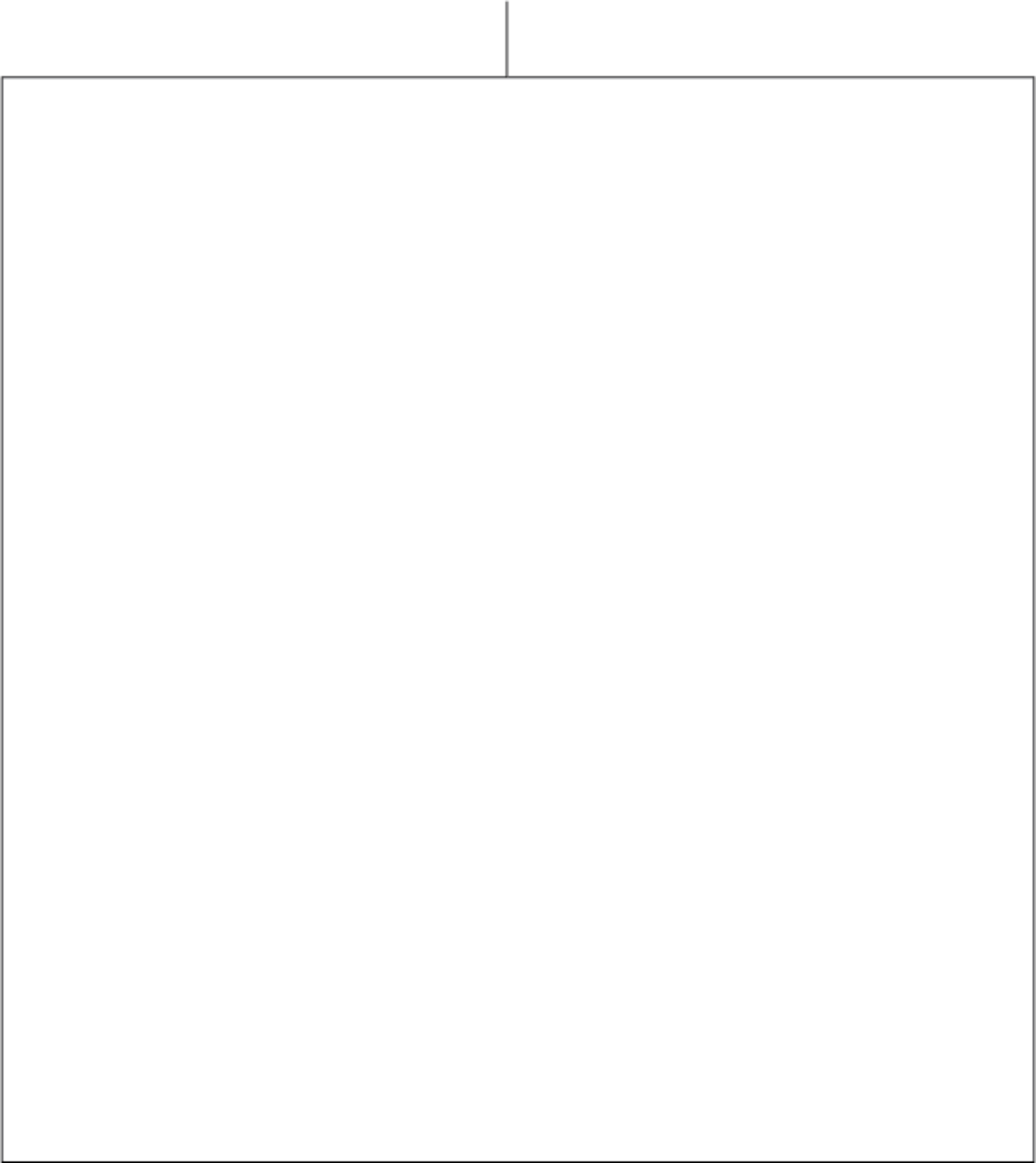A rectangular box with a thick gray border is depicted against a white background, positioned in a portrait orientation. The box is slightly taller than it is wide, akin to the dimensions of a lung, and it contains no text, images, or any form of information. At the top center of the rectangle, extending vertically upwards from its middle, is a thin vertical line. The interior of the box is completely blank, suggesting it could serve as a frame or placeholder for content that is currently missing. Despite its usual function to contain some form of detail, the box remains void of any descriptive elements, leaving its purpose ambiguous.